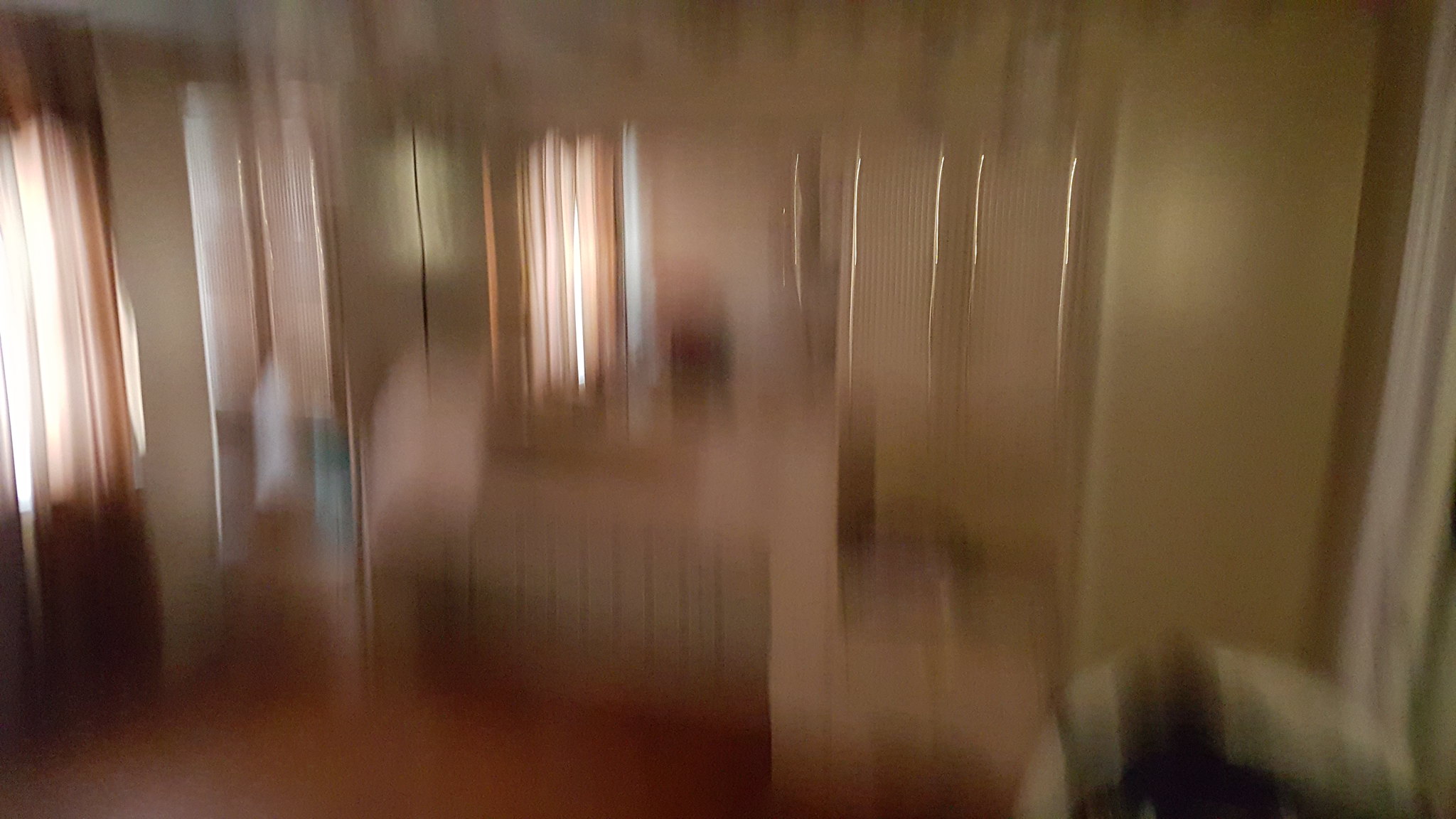This photograph, though extremely blurry, appears to depict a spacious bathroom or spa-like setting. The room features cream-colored tile work intertwined with walls adorned in pinstripe wallpaper, which gives the space a unique visual texture. The pinstripes reflect light, creating long, shiny lines across the walls. On the left side of the image, natural light streams through a window covered by sheer curtains with a rust-colored border, adding a warm, inviting touch to the ambience. Toward the back, there seems to be a walk-in shower or possibly a combination walk-in sauna and shower, enhancing the luxurious feel of the space.